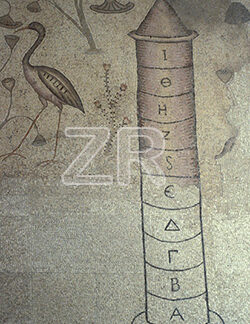The image appears to be a grainy photograph of a hand-drawn illustration, featuring dark and unclear lighting conditions that make the colors hard to discern, leaving a predominant gray tone. Central to the composition is a narrow, segmented tower resembling a rocket or a silo with an inverted cone at the top. Each segment of the tower contains a unique letter: starting from the top, there is an I, followed by O, H, Z, S, E, a delta symbol, a Cyrillic letter R, B, and A at the bottom. On the upper left corner of the page, a crane or ibis is depicted eating from conical flowers, set against a backdrop of a flowering shrub and a tree. Additionally, the image features prominently centered white lettering that spells out "ZR." The overall scene suggests a juxtaposition of natural elements with symbol-laden architectural or mechanical structures.